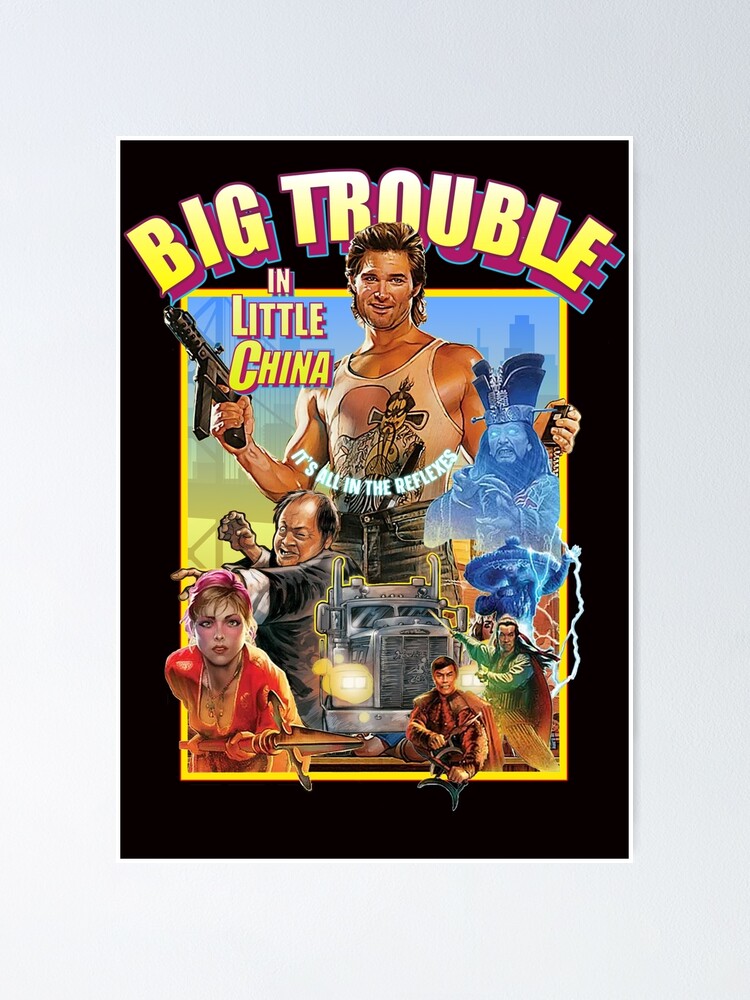This movie poster for "Big Trouble in Little China" is prominently displayed on a white wall. The background of the poster is black, accented with bold yellow lettering outlined in purple at the top that reads "Big Trouble in Little China." The tagline "It's all in the reflexes" is also featured on the poster.

Centrally positioned is the main character, likely played by Kurt Russell, dressed in a tank top with a design, black jeans, and wielding a machine gun. He is also holding an ambiguous object in his other hand. Surrounding him are various other characters: an imposing Asian man with a large hat and glowing eyes, another hidden-faced figure with a big hat, and a long-haired Asian individual in a green top and yellow pants.

At the bottom center of the poster, there is an image of a Mack truck with its lights on. To the left, a female character with blonde hair is dressed in red, including a red hat, and brandishing a spear-like weapon. Adjacent to her is an older, slightly balding Asian man, clad in a black robe with white accents, seemingly engaged in combat with his hands.

The poster is brimming with vibrant colors, including various shades of blue, yellow, orange, red, and silver, concentrated in the center. Additional elements include a man in a black jacket, a girl with a gold necklace and pink hair holding a sword, and a spaceship surrounded by white lightning bolts, making the poster a vivid and intricate depiction of the film's eclectic cast and dynamic action.